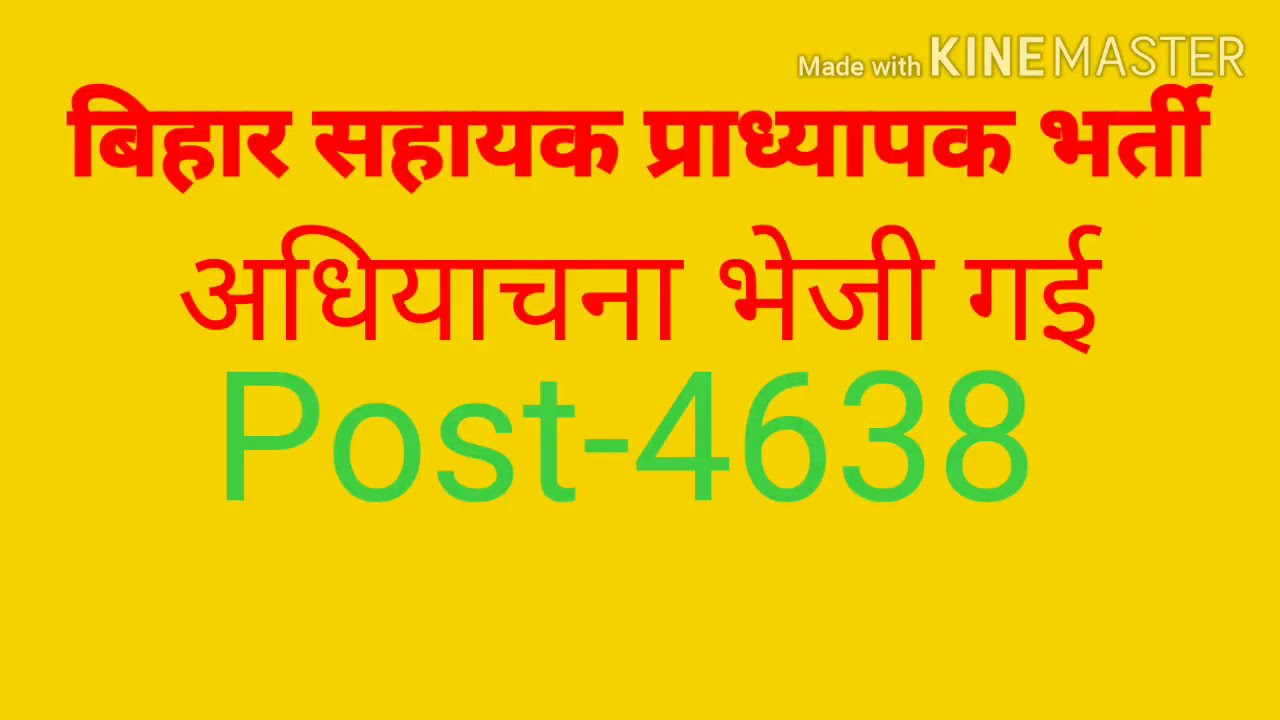The image features a rectangular, bright yellow background with various inscriptions. In the upper left corner, "MADE WITH" is written in a whitish off-white color, followed by the words "KINE MASTER" in larger, all-capital letters. Below this, there are two lines of bold, red text written in an unidentified Middle Eastern script, possibly Arabic. The first line features block letters, while the second line consists of skinnier, taller letters. At the bottom, in a bluish-green color, the word "POST" is displayed, followed by "P-4638" in the same color. The text suggests this might be an advertisement or a social media element.